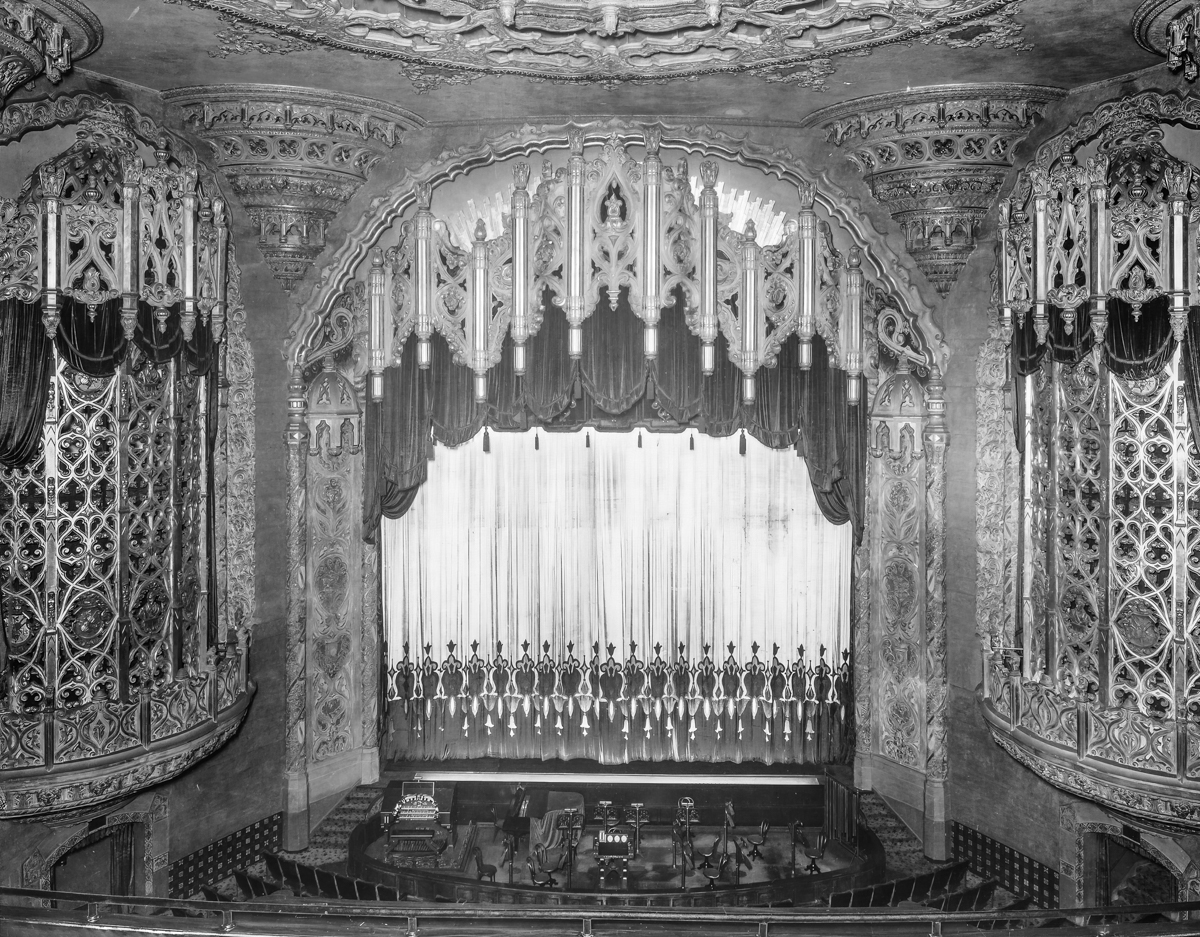This black-and-white photograph captures the grandeur of an old, opulent theater, renowned for its classical music performances. The perspective appears to be from the mezzanine or a couple of floors up, looking over the empty, elegant seats of the orchestra floor towards a stage adorned with intricately designed metal railings and a large arch that stretches to the high, beautifully detailed ceiling. The stage, currently unveiled with the curtain pulled up, reveals an orchestra pit with various instruments, possibly including an organ and a piano. Both sides of the theater feature luxurious, domed balconies, likely reserved for affluent patrons, adding to the venue’s pompous aesthetic. These sections are gated with ornate, nature-inspired designs and heart-shaped motifs that are especially opulent. The rich architectural details and artistic elements throughout the theater emphasize its historical and cultural significance, captured timelessly in this monochromatic image.